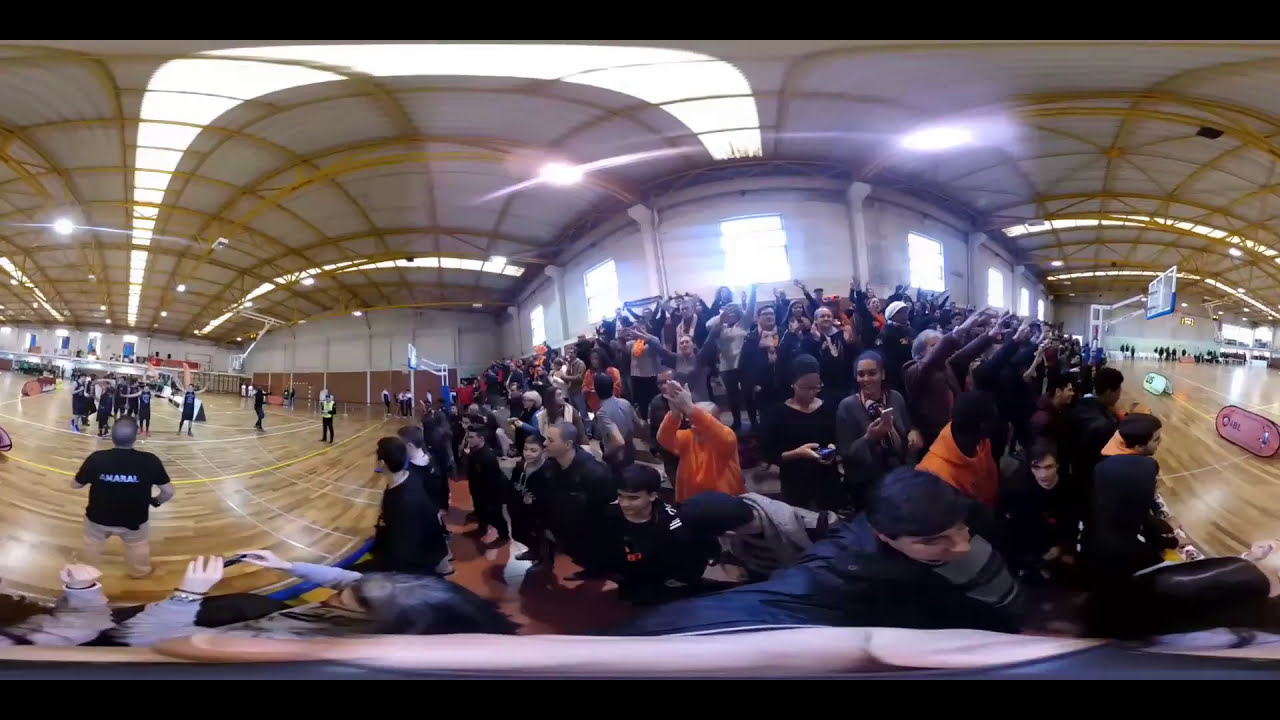The image depicts a detailed, 360-degree panoramic view inside an indoor sports hall, likely during a daytime event evidenced by sunlight streaming through the windows. At the center, a diverse crowd of spectators, including men and women of different races, are visible, some standing and cheering with their hands in the air. The crowd is dressed in various attire, with some individuals in black clothing, possibly team supporters, and orange shirts scattered among them. There is an evident security presence around the gym court, where the event is taking place.

On the left side of the image, players in black jerseys and shorts, indicative of a basketball or volleyball team, are gathered near the basketball hoop and backboard. The gym floor, made of light wood and marked with yellow and white lines, hints at multiple sports activities.

To the right, the picture encompasses another section of the court, distinguished by cylinder-shaped popup banners along its edges, though no active game play is observed in this area. The ceiling structure features notable metal yellow beams and transparent curved windows that run the length of the sports hall, enhancing the bright and open feel of the space.